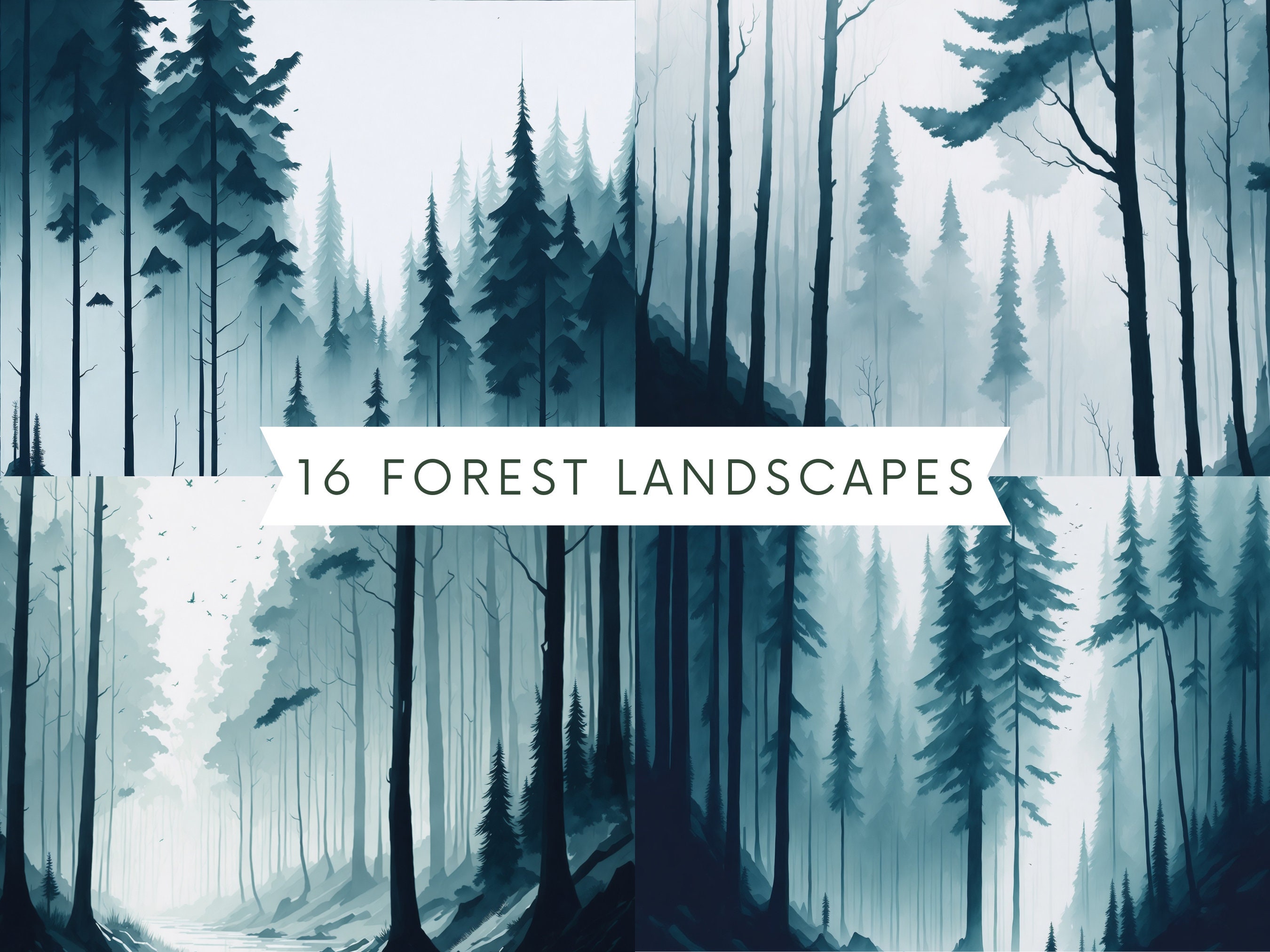The book cover, titled "16 Forest Landscapes," features a detailed black and white sketch with a subtle but distinct greenish-grey tinge. The cover is divided into an upper and lower section, each portraying a forest landscape with tall pine trees, dark in the foreground and fading into shadowy, faint ones in the background. The scenes evoke a slightly foggy atmosphere with tinges of blue and green, adding an artistic appeal rather than lifelike colors. Situated across the center of the cover is a white banner with clipped ribbon ends, bearing the title "16TH SPACE FOREST" in bold black capital letters. The imagery on the cover focuses on the various forest scenes, emphasizing the diverse textures and hues of trees under different conditions.